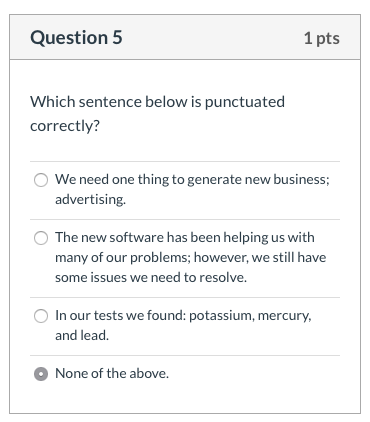The image features a rectangular layout with a distinct color scheme and structured sections. The overall rectangle is blue on the left side, while the top, right, and bottom borders are grey. Positioned at the top of this rectangle is a grey rectangle labeled "Question 5" on the left and "1 PPS" on the right. Below this label, a grey line divides the header from the main content.

The content beneath poses the query, "Which sentence below is punctuated correctly?" This question is separated from the answer choices by another grey line. Following the question are three multiple-choice options, each housed within a grey outlined circle, and a final option within a highlighted selection circle. 

The first grey outlined circle contains the sentence, "We need one thing to generate new business: advertising." 

The second grey outlined circle presents the sentence, "New software has been helping us with many of our problems: however, we still have some issues we need to resolve." 

The third grey outlined circle offers the sentence, "In our tests we found: potassium, mercury, and lead." 

The fourth and final option is a grey outlined circle with a concentric white circle inside it, labeled "None of the above."

All the text within these sections appears in blue, maintaining a consistent visual theme throughout the image.